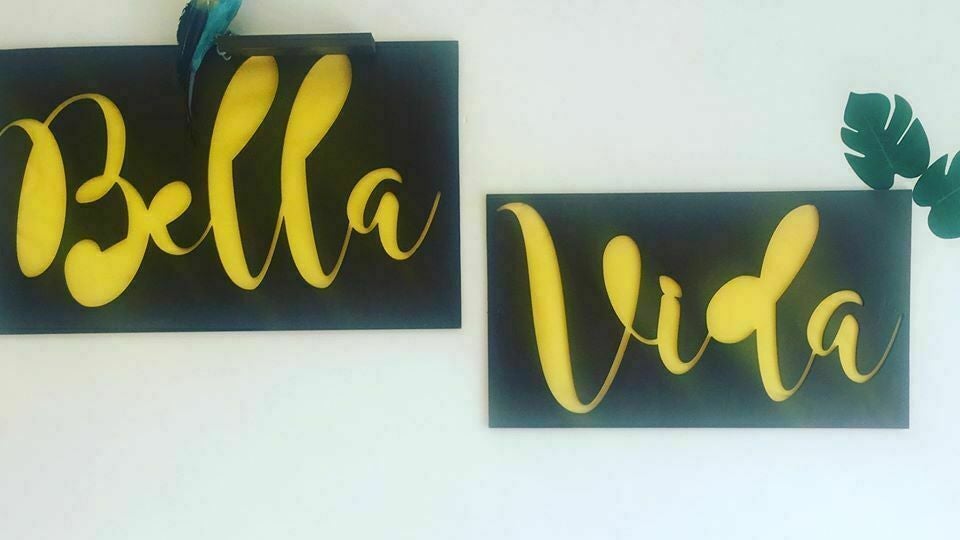The image displays a detailed and artistic scene featuring two distinct rectangular signs set against a soft, mint green background. The sign in the top left corner reads "Bella," with yellow letters on a black background, and is adorned with a vibrant blue bird perched atop it, showcasing bright blue body feathers and darker tail feathers. The sign in the bottom right corner, a bit lower and towards the center, reads "Vida" and is complemented by two green leaves with slits on their upper right corner. The overall arrangement suggests an artful, playful environment, possibly in a child's bedroom or an art studio, illuminated by natural light that enhances the clarity and color contrast, displaying various hues such as off-white, light blue, black, yellow, turquoise, and green. The combined elements and the thematic typography evoke a whimsical sense of "Bella Vita," meaning "Beautiful Life."